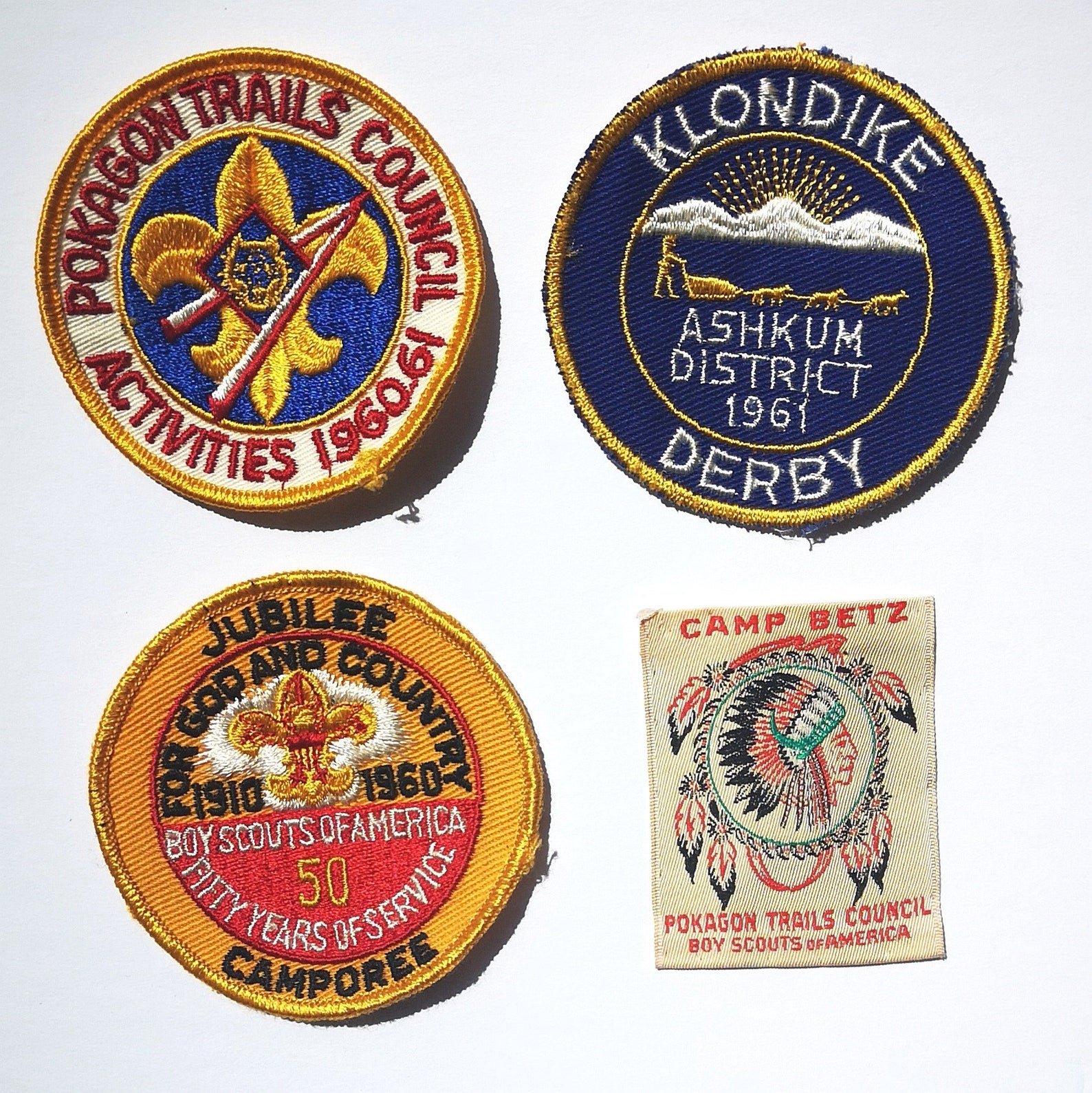The image showcases four distinct Boy Scout patches, emblematic of various activities and commemorations. 

In the top left, a round patch from the Pokégon Trails Council Activities 1960-61 features a gold Fleur de Lys on a blue background. Adjacent to it, the top right patch is also circular with a blue and gold trim. This badge, from the Klondike Ashcombe District 1961 Derby, depicts a sun rising over mountains and a man behind a dog sled with three dogs. 

On the bottom left, another circular patch, this one predominantly orange, celebrates the Boy Scouts of America's 50th Anniversary Jubilee for God and Country 1910-1960, with a gold Fleur de Lys and the text "50 years of service." 

The final patch, located on the bottom right, is square and primarily white. It features an image of a Native American chief's head adorned with feathers, encircled by a Dreamcatcher-like motif. The text reads Camp Betts, Pokégon Trails Council, Boy Scouts of America. 

These patches collectively highlight significant events and milestones within the Boy Scouts organization.